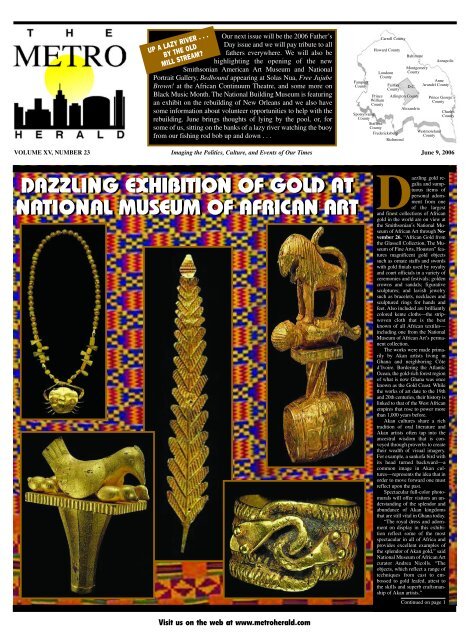This image depicts the cover of a Metro Herald magazine dated June 9, 2006, Volume 14, No. 23. The top left corner prominently displays the Metro Herald logo. Just below this, a small article is presented in white text against a black background. On the top right, there is a simplified map of the Washington D.C. metro area.

The main section of the cover, occupying the lower portion, features a dazzling exhibition at the National Museum of African Art. The background is black, with vibrant orange and blue patterns framing the various segments. Showcased are several intricate golden artifacts, including necklaces, statues, pendants, and a bracelet, all reflecting the rich heritage of African art. Decorative African colors and art styles enhance the visual appeal around these images. On the right-hand side is a vertical text box containing additional information, which mentions that the article continues on the next page. Along the bottom of the cover, a website address is visible, further connecting readers to more details. The overall image quality appears to be poor, slightly obscuring some finer details.